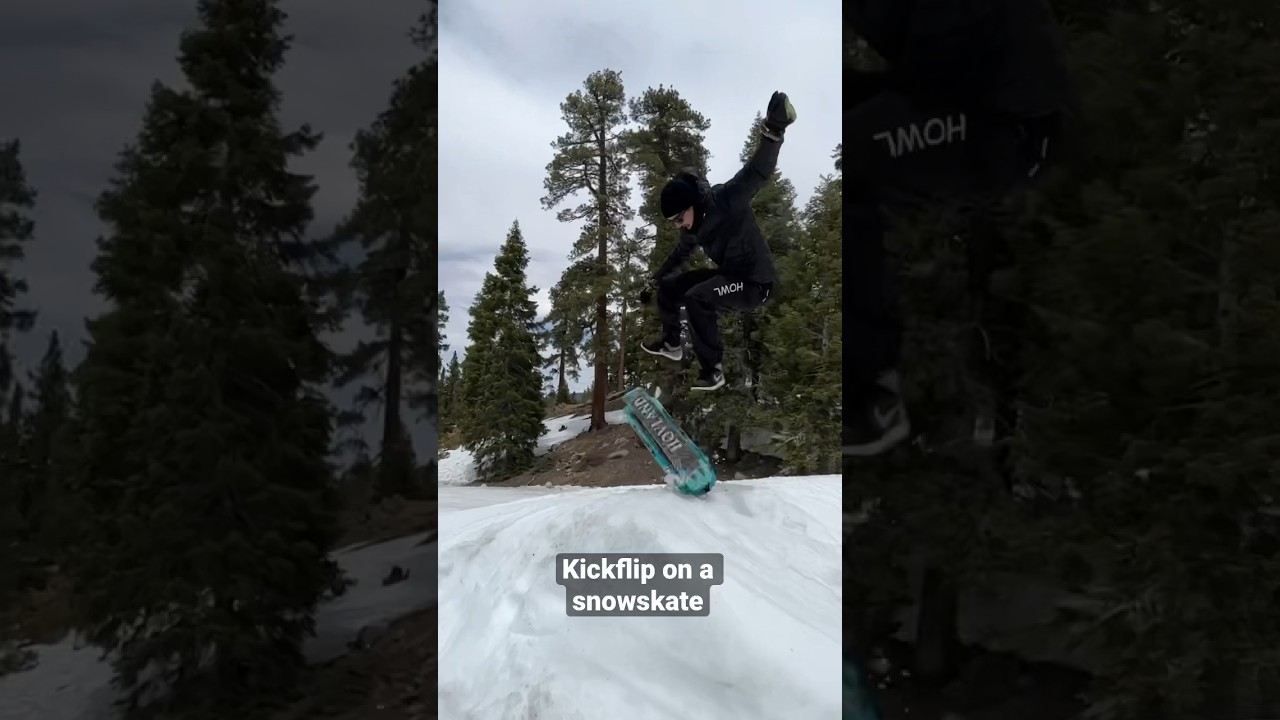The image presents a composition that resembles a collage with three distinct segments. Both the left and right portions of the image are darkened and appear to be expanded versions of the central, smaller picture. This central image depicts an outdoor scene with a man executing a kickflip on a snowskate amidst a snowy landscape. The man, clad entirely in black, is captured mid-air with his green snowskate. The background features an array of Christmas trees and other trees, with patches of snow and exposed dirt on the ground, indicating light snowfall. The sky above him is partly cloudy. Along the bottom of the image, white text reads "kickflip on a snowskate," highlighting the man's acrobatic maneuver.